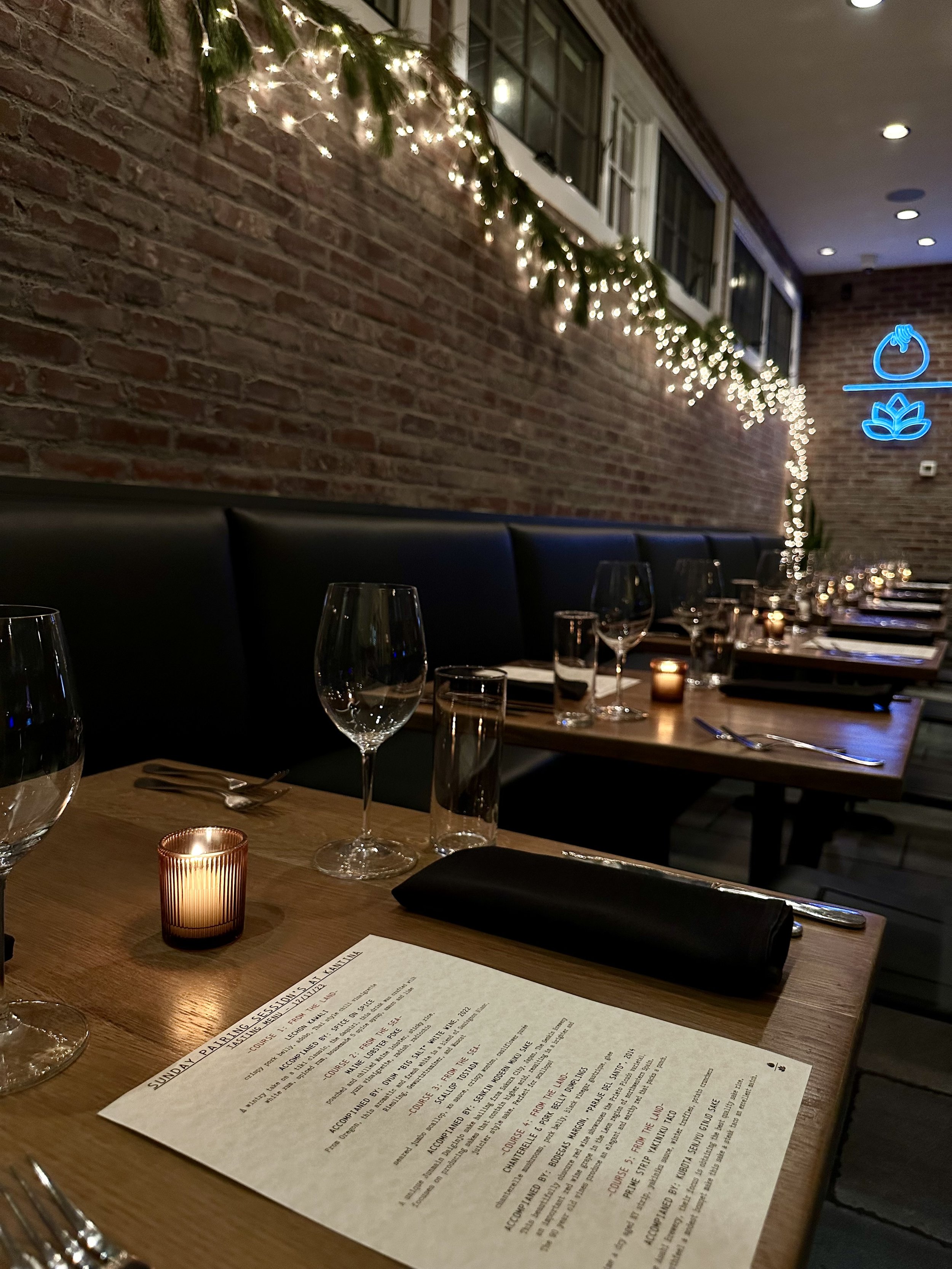The image depicts a stylish, upscale restaurant characterized by its intimate and ambient lighting. The restaurant features a row of black leather or vinyl booths situated on the back left, accompanied by small, square wooden tables arranged neatly in front. Each table is meticulously set with a lit tea light candle, a pair of wine glasses, smaller water glasses, silverware, and a rolled-up black napkin. A paper menu with black text – detailing the "Monday pairing sessions at Cantina" and listing gourmet dishes like Maine Lobster Poke, Scallop Tostada, Pork Belly, and Prime Strip Taco – rests on each table. The menus indicate a recent date, 12-17-23. The decor is enhanced by Italian string lights running along the top of a brick facade with high windows and embedded round ceiling lights. At the end of the row of tables, a bright turquoise blue neon sign resembling a plant symbol adds a modern touch to the rustic brick interior. The ambiance suggests a high-end, trendy dining experience.